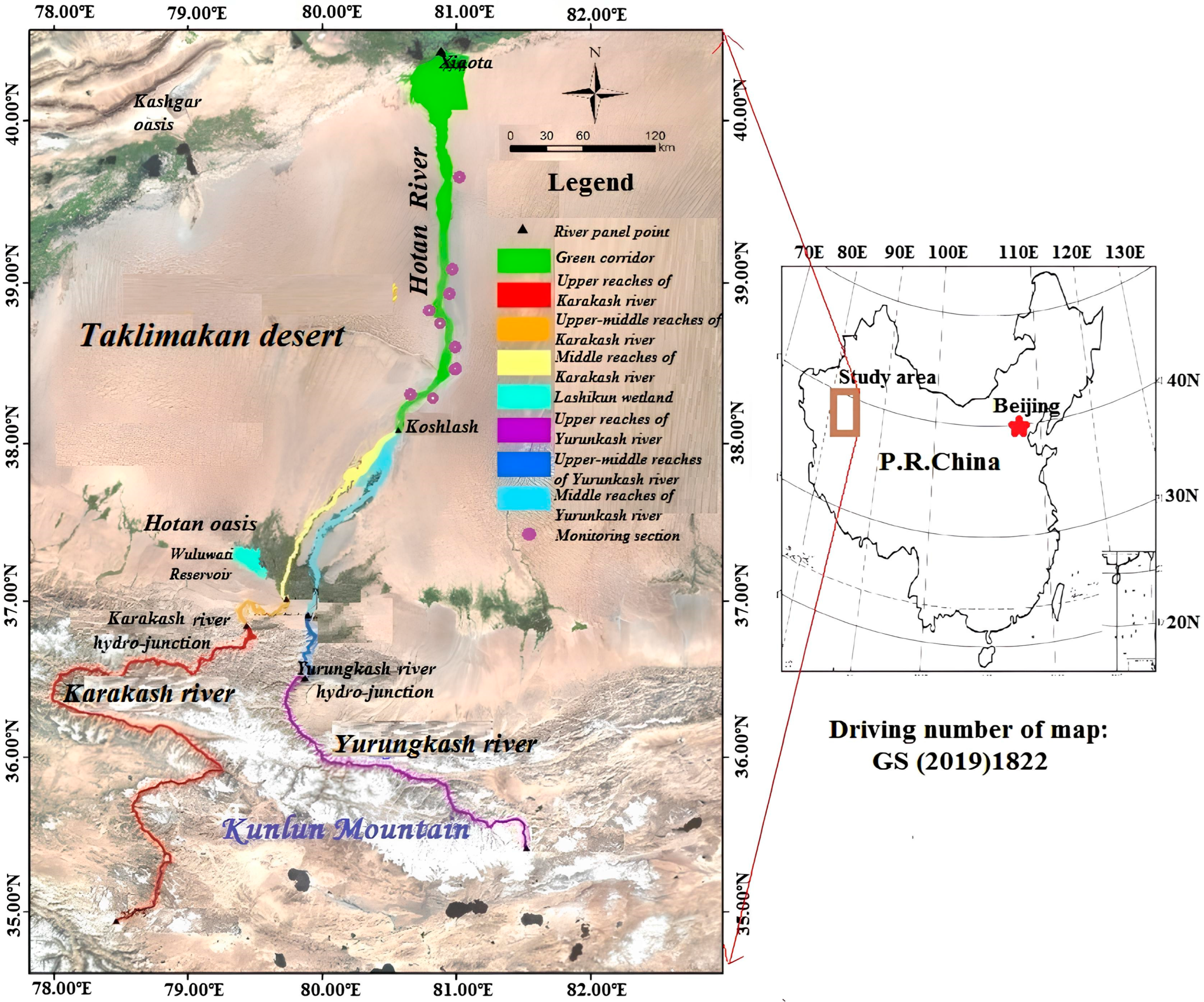The image features two maps side by side. On the left, there is a detailed, color-coded map focusing on the Taklamakan Desert, highlighting various features and river sections. The map is meticulously labeled with elements such as the Green Corridor, upper, middle, and lower reaches of the Karakash River, and similar segments of the Uran Kash River. It shows a variety of geographical features including two oases, a hydro junction, and a reservoir. The map's colors range from green, red, orange, yellow, and shades of blue to purple, each representing different river segments traversing the desert. A legend and scale bar (ranging up to 120 kilometers) provide additional context, while a compass rose is positioned in the upper right corner. Latitude and longitude degree markers are noted along the map's perimeter for precise location referencing.

On the right, a smaller black and white map labeled "PR China" shows an outline of China on a globe projection with latitude and longitude lines. Beijing is marked with a red star. A brown-outlined rectangle labeled "Study Area" indicates the region highlighted in the detailed map to the left. The right map also includes detailed coordinates and mentions the driving number of the map: GS20191822.